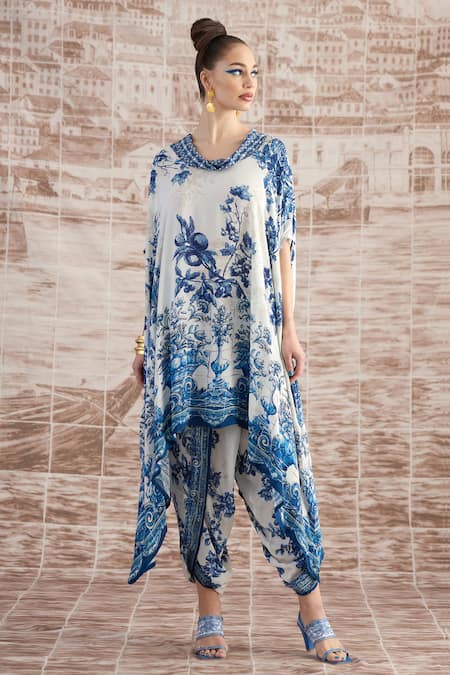This vertical color photograph captures a striking fashion model, who exudes an almost surreal quality with her tall, slender frame and plastic-like skin texture, suggesting a digitally enhanced or Photoshop-conceived image. The model, poised and elegant, gazes towards the upper right corner of the photograph.

She wears a stunning long sari garment paired with baggy pants, both adorned in a delicate white fabric detailed with intricate dark blue and light blue floral patterns reminiscent of fine china designs. Her ensemble is completed with strappy, high-heeled sandals featuring thick strips of fabric that elegantly cross her feet. 

The background is a sepia-toned fabric cloth, depicting an ethereal scene of a river and light pastel buildings, adding a dreamlike quality to the composition. The entire setting evokes a sense of timeless elegance, blending traditional clothing with a modern, almost otherworldly fashion statement.